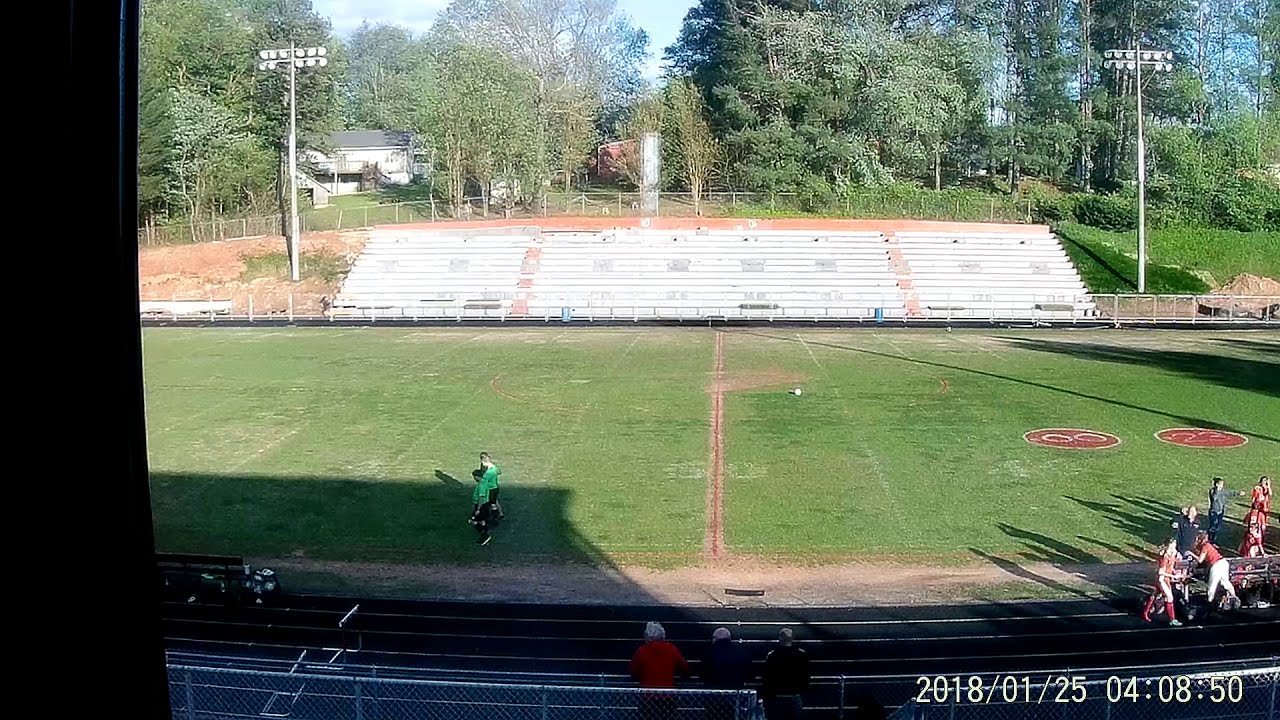The image captures a football stadium repurposed for a soccer game on a sunny day. The field, vividly green, still displays faint white yard lines and a distinct 50-yard line marked with a red stripe. In the foreground, there's a running track encircling the field, bordered by a fence and the bottom of the home stands. The background reveals the visiting team's metal bleachers under bright sunlight, with two light posts adjacent and a fence line framing trees and houses. The photograph appears to be taken from inside a building, as the dark window frame is visible on the left. On the 45-yard line to the left stand two referees donning green tops and black shorts. Scattered across the lower right corner and along the track are soccer players in red and white uniforms and others in gray and black. Additionally, three spectators, clad in red, blue, and black jackets, overlook the field from the foreground stands. The image is timestamped 2018-01-25 04:08:50 at the bottom right corner.